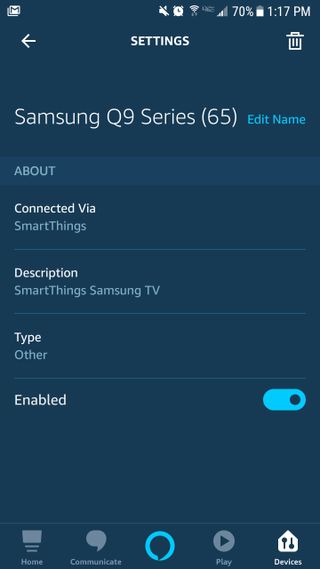This screenshot, captured from a smartphone, prominently displays a variety of interface elements and system status indicators. In the top left corner, the Gmail icon is visible, while the top right corner features icons for sound off, alarm, Wi-Fi, network coverage, and battery charge, which is at 70%. The time is displayed at 1:17 p.m.

Centered at the top of the screen is the word "Settings," with a trash bin icon immediately to its right. Below this header, the text "Samsung Q9 series (65)" is displayed, indicating the specific model name of the device. This text is accompanied by an option to edit the name. Directly underneath, there's a section labeled "About," and beneath that, another piece of text reads, "Connected via SmartThings."

Further detailed information includes a description: "SmartThings Samsung TV." The type of device is categorized as "Other," and the enabled status is switched on.

At the bottom of the screenshot, five icons are arranged from left to right: the Home button, the Communicate button, a central blue circle (likely indicating a key navigation action), the Play button, and finally, the Devices button located in the extreme bottom-right corner.